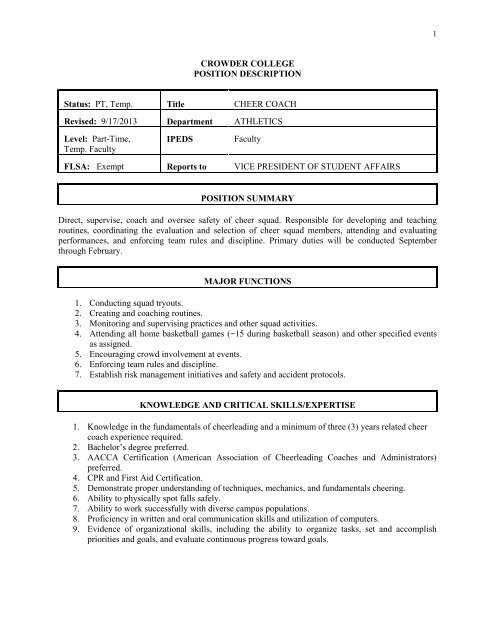The image depicts a formal, text-based document resembling an 8x10 or 11x14 sheet of paper with a white background and black text. At the top, the centered header reads "Crowder College Position Description." Below this is a bordered rectangular area featuring two columns. The left column includes details like "Status: PT Temp," "Revised: 9-17-2013," "Level: Part-time Temp Faculty," and "FLSA Exempt." The right column provides specific job details: the "Title" is "Cheer Coach," the "Department" is "Athletics," the "Reports To" field names the "Vice President of Student Affairs."

Below this bordered rectangle, a thin rectangular section labeled "Position Summary" describes the job, emphasizing the responsibilities of direct supervision, coaching, and overseeing the safety of a cheer squad. Further down, the header "Major Functions" introduces a numbered list from one to seven, detailing various duties such as coaching the cheer squad and creating routines. The section below this, titled "Knowledge and Critical Skills," outlines nine required expertise areas, including knowledge of cheerleading fundamentals and a minimum of three years of related cheer coaching experience.

The document is structured in a clear, formal style and appears to be a printed job description for a position at Crowder College.